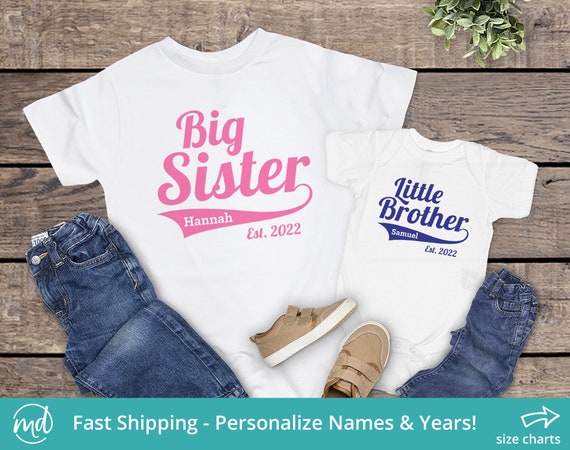The photograph showcases an advertisement for family-themed clothing, centered on a set of two white t-shirts and two pairs of blue jeans. Positioned on a wooden, horizontally slatted background, the larger t-shirt on the left features the text "Big Sister Hannah, EST 2022" in pink cursive letters, accompanied by a swish mark with the name. To the right is a smaller, similarly styled t-shirt that reads "Little Brother Samuel, EST 2022" in blue cursive letters. Flanking the t-shirts are two pairs of blue jeans, with the larger pair to the left and the smaller pair to the right. A pair of brown shoes with a white base is placed centrally at the bottom of the image. To the lower section, blue text advertises "MD" in a circle, "fast shipping, personalized names and years" with an arrow pointing to "size charts." Adding a touch of nature, a potted plant with green leaves is located in the top right corner, enhancing the overall fashion-forward, family-centric setting.